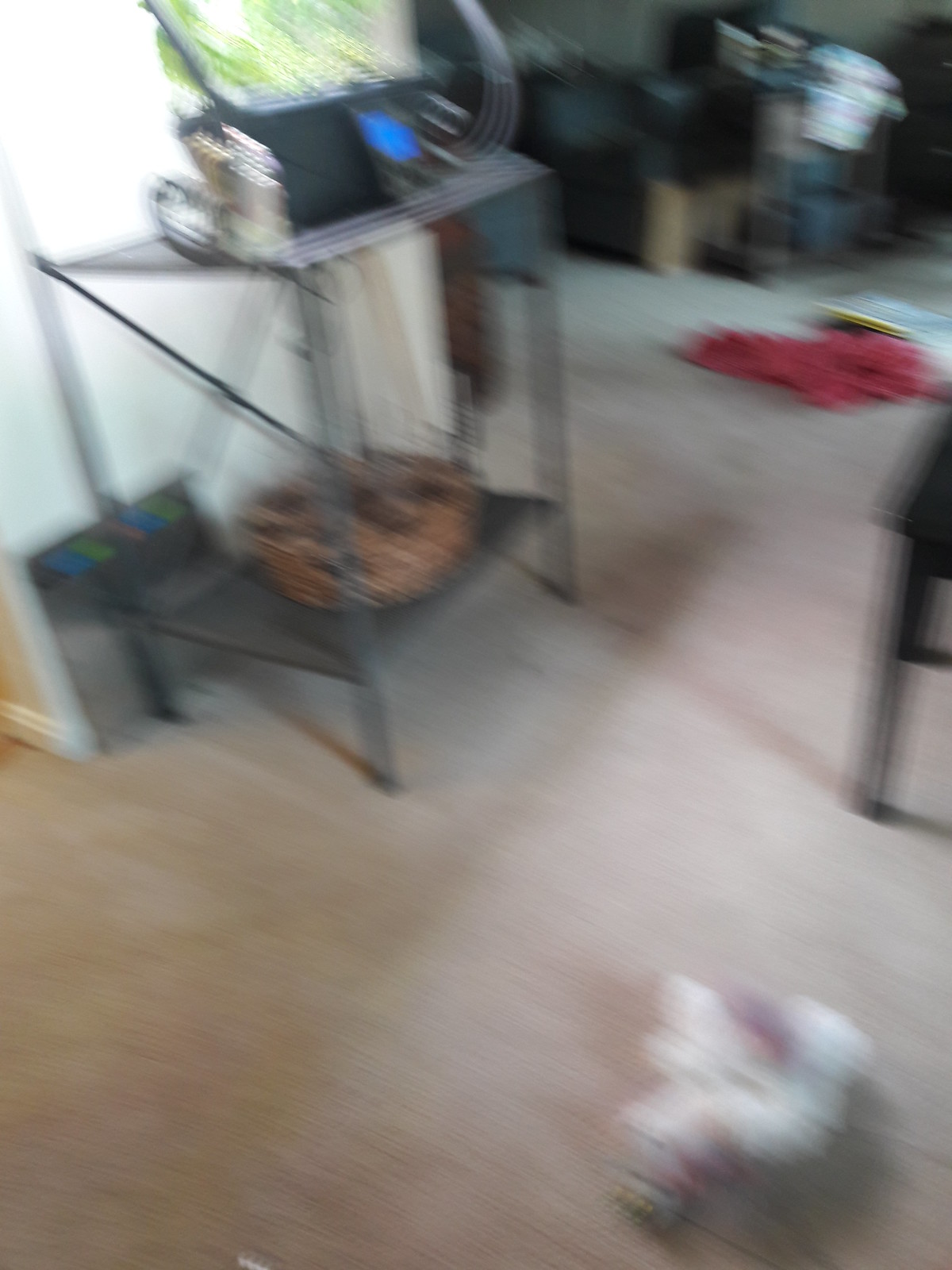This is a blurry photo taken inside someone's living room. The home features a beige-colored carpet with scattered items and clutter. In the center of the photograph is a silver, square-shaped metal stand, possibly a wrought iron table. The stand has a lower shelf, which holds a wooden basket, and the top shelf appears to have an aquarium with a black base and illuminated green foliage inside, though it's hard to discern details due to the blurriness. To the right, there's an armchair, with a difficult-to-identify person, possibly sitting. On the floor near the chair are various items, including red clothing and something white and pink. Additionally, the top right corner shows some boxes and more clutter against the wall. The wall on the left of the photo has a visible white vent and a turn leading into a hallway.